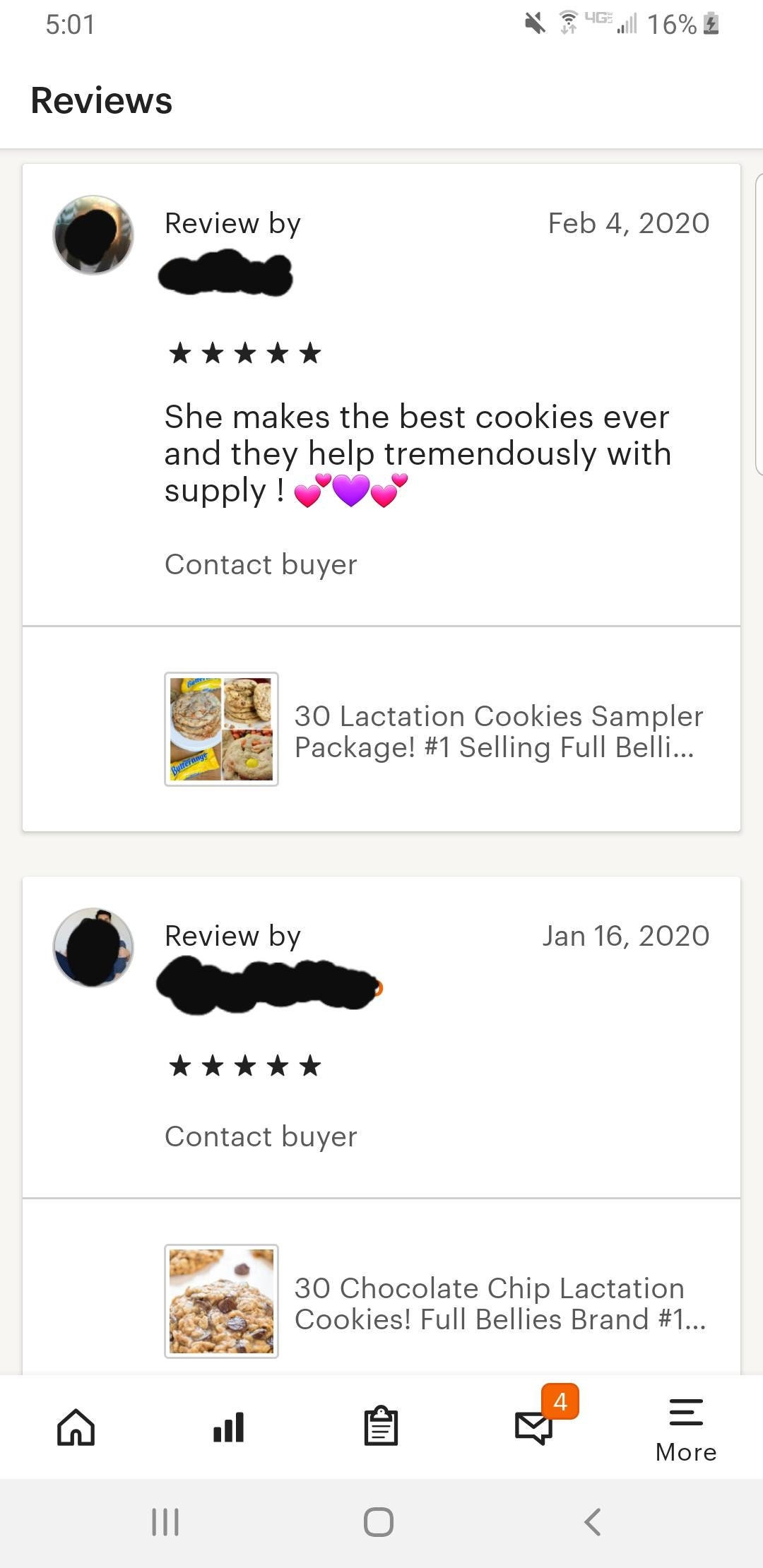The image showcases a smartphone screen displaying a detailed review page for a product, specifically "Dirty Lactation Cookies." The top of the screen includes typical smartphone indicators such as the time (5:01), battery percentage (16%), and battery icon, providing a sense of real-time viewing.

Immediately below, the screen headline “Reviews” introduces the content. The review section prominently features two distinct reviews within a long rectangular box. The identifiers of both reviewers are censored, maintaining their anonymity.

The first review, dated February 4th, 2020, is rated five stars. The anonymous reviewer praises the product enthusiastically, stating, "She makes the best cookies ever, and they help tremendously with supply!" This review includes decorative elements such as pink and purple heart emojis. Adjacent to the review is an option to "contact buyer," adding an interactive element.

Beneath the first review, the product detail reads "Dirty Lactation Cookies Sampler Package Number One," accompanied by an image of the cookies, suggesting a visually appealing product presentation.

The second review, dated January 16th, 2020, also carries a five-star rating. This feedback highlights "Dirty Chocolate Chip Lactation Cookies," tagged under "full bellies, brand number one." Similar to the first, the option to contact the buyer is available and an image of the cookie is present to entice potential buyers.

At the very bottom of the screen, standard phone interface icons are displayed: home, data usage, calendar, email with four unread messages, and a “more” option symbolized by three lines. Additional navigation icons such as an arrow pointing left and a square are visible, likely serving as back or home functions.

Overall, the captured smartphone screen offers an organized and visually appealing layout of customer reviews, emphasizing the positive feedback and interactive features for a product-based application interface.